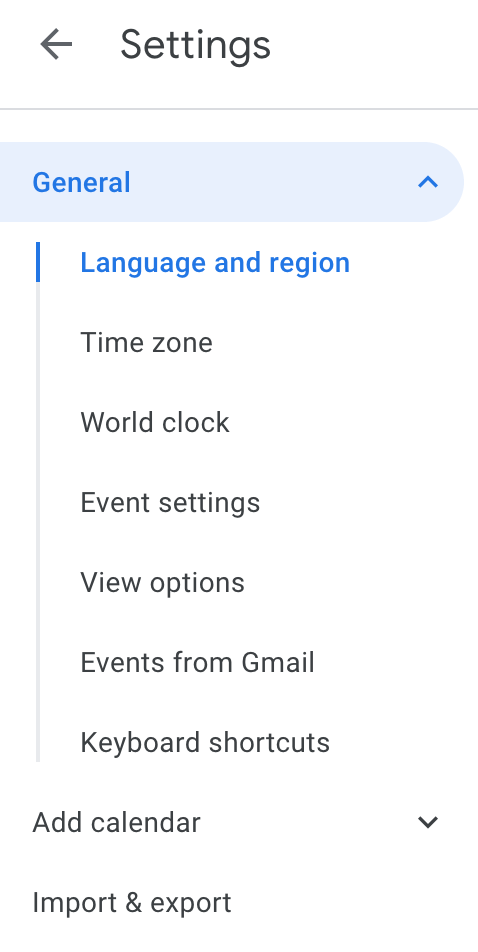This screenshot displays a vertical filter/menu section from a website or application resembling a Google-designed interface. The layout suggests a settings sidebar or pop-out menu on a predominantly white background. The top of the sidebar features the word "Settings" in sans-serif font, accompanied by a left-pointing arrow, below which lies a thin gray separator line. 

Directly underneath, there's a light blue rectangular area with rounded edges, labeled "General" in blue text, and marked with an upward arrow. This signifies the primary menu section, within which several submenu options are listed: "Language and Region," "Time Zone," "World Clock," "Event Settings," "View Options," "Events from Gmail," and "Keyboard Shortcuts." These submenus are demarcated by a light gray vertical line on the left, with the "Language and Region" option highlighted in blue, indicating it is currently selected.

Further down, additional primary menu options include "Add Calendar" and "Import and Export." The absence of any visible mobile or browser UI elements suggests that the screenshot captures only the content section of the website or application.